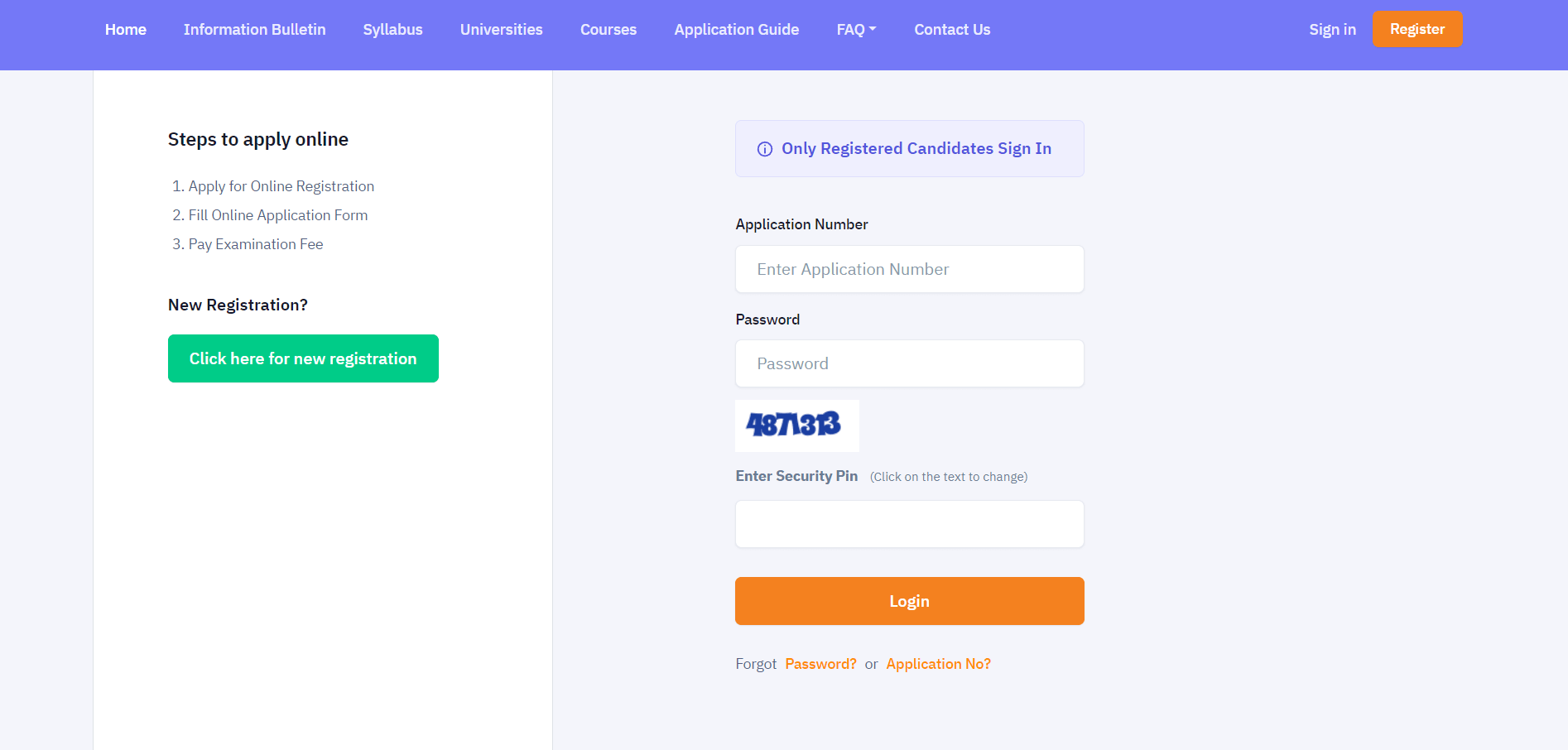This image is a screenshot of a website designed for online registration and application. The screenshot is rectangular, with the top and bottom edges being longer than the sides. 

At the very top, there is a prominent light blue banner that spans the entire width of the page from the left to the right. This banner contains several lines of interactive white text, each serving as a link to different sections of the website. Starting from the left, the clickable links are labeled "Home," "Information Bulletin," "Syllabus," "Universities," "Courses," "Application Guide," "FAQ," and "Contact Us." Towards the top right corner of this banner, there is additional interactive white text that reads "Sign In." Next to it, there is an orange rectangle with rounded corners featuring white text that says "Register."

The primary background color of the remainder of the page is light gray. The bottom of the page is divided into two sections: a white banner on the left and a login area on the right with multiple input boxes.

The white banner on the left side contains black text detailing the steps for online application. The steps are listed as follows:
1. Apply for online registration.
2. Fill online application form.
3. Pay examination fee.
Below these instructions, there is a green rectangle with white text that prompts users to click for new registration.

On the right side, the login area comprises several input boxes with a white background and gray placeholder text, guiding users on where to enter their login information.